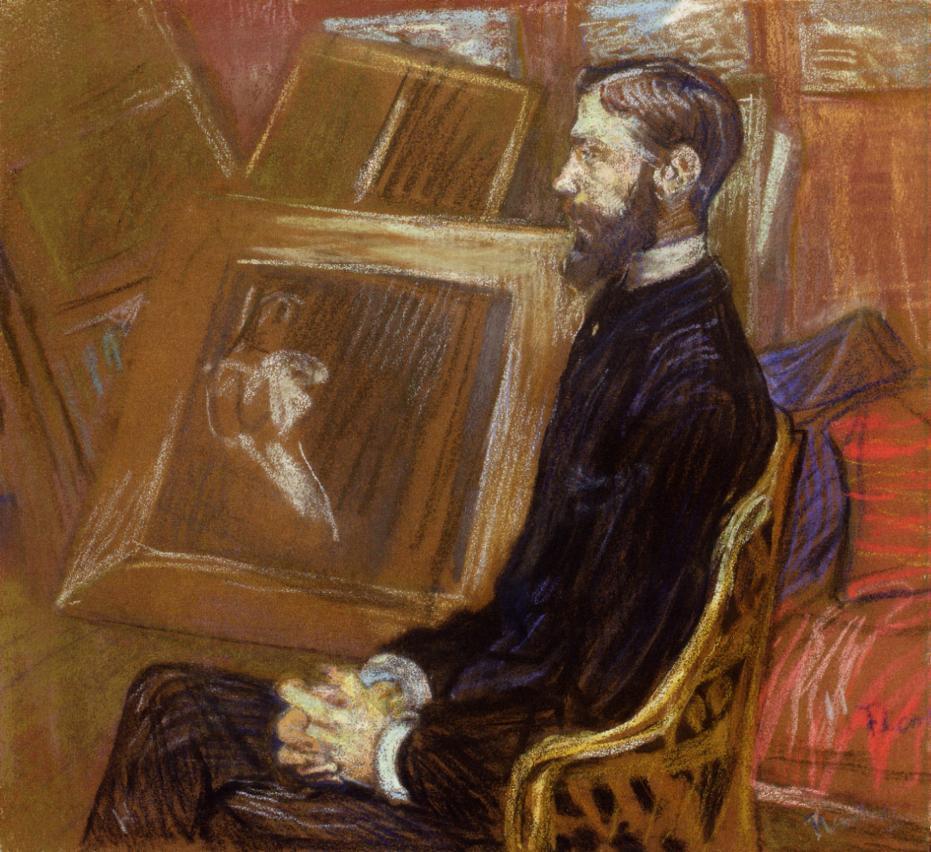This detailed pastel drawing features a tall, thin man with a short brown beard and a mustache, seated in a gold-colored, ornate wooden chair. The man, who appears to be of European Caucasian descent, faces towards the left with a serious expression. He is dressed in an all-black long-sleeved shirt with subtle pinstriping, over a white undershirt that reveals its collar and sleeves. His pants are a dark shade, either black or dark gray. The man's right leg is crossed over his left, and his hands are clasped together, resting in his lap. The background is abstract and colorful, featuring a variety of squares in blues, grays, and pinks, especially vibrant on the right side. Additionally, the back wall is adorned with an assortment of empty picture frames in gold and yellow, stacked together. Behind the man, there appears to be a couch or bed-like structure draped in red and purple.